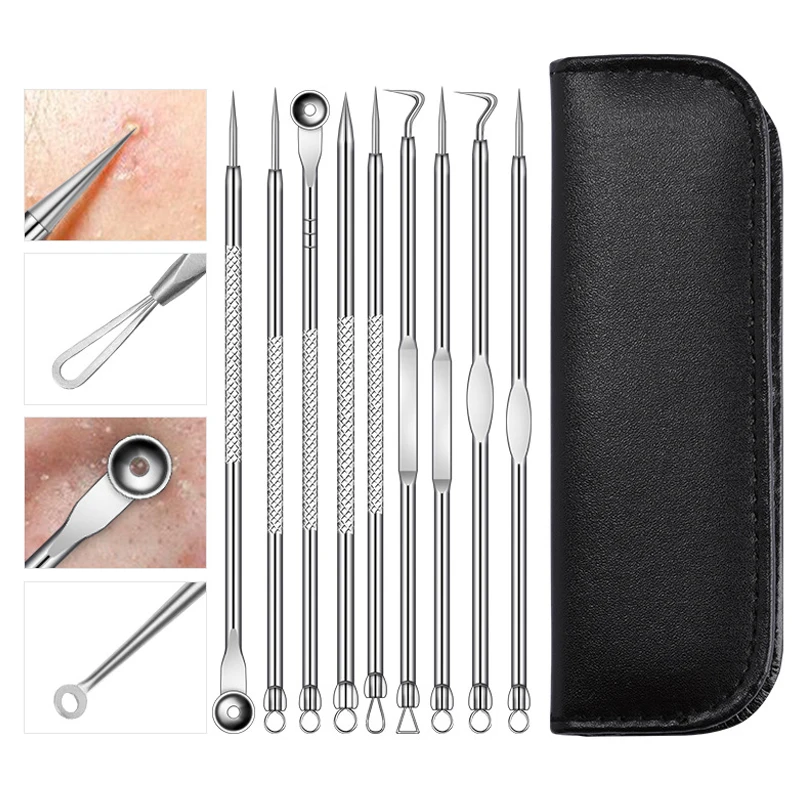The image depicts a complete comedone extractor tool set, designed for skincare purposes such as extracting blackheads, pimples, and other blemishes. The central part of the image prominently displays nine long silver instruments, each featuring various pointed and looped tips tailored for different forms of skin extraction. The tools come neatly stored in a black leather case seen on the right side of the image. The left side of the image contains a series of four magnified inset photos, illustrating the usage of these tools on blemished skin or highlighting the detailed designs of the tool tips. The background is plain white, implying that this is a catalog or webpage listing. The close-up images emphasize the precision and care needed when using these sharp, metal instruments.